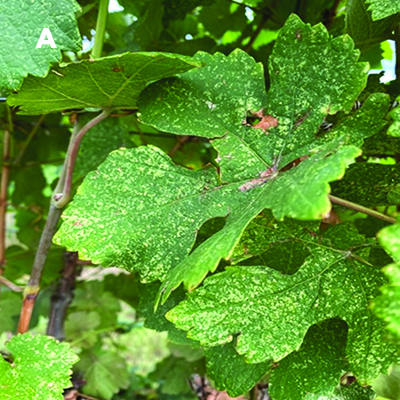In this square photograph taken during daytime, we see an intricate close-up view of several vibrant green elm leaves. The main focus is on four or five leaves with a lush green background, likely composed of similar elm leaves and branches. In the upper right corner, the letter 'A' in white subtly overlays one of the leaves.

The primary leaf, which is centered in the image, exhibits signs of having been nibbled on, with a distinct round hole in the upper left section, bordered by brown, indicating the area where the leaf was eaten. The leaf's surface shows no visible insects but contains some light specks, which might suggest a minor disease or could simply be a normal characteristic of the leaf. 

The leaves display a slight yellowish edging, while the deeper inner green contrasts beautifully with the white veins running through them. The slender stem attaching the leaf to the tree is a light golden brown. Through the gaps between leaves and branches, bits of blue sky peek through, adding a serene touch to this detail-rich photograph.